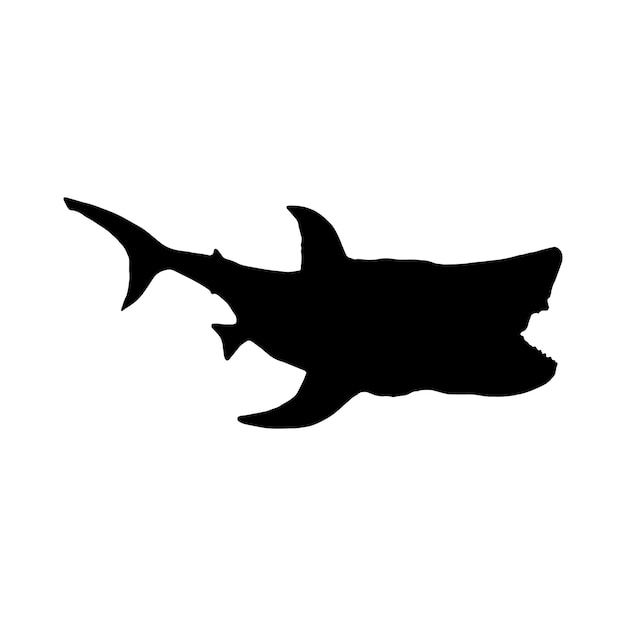The image is a detailed, black silhouette of a marine creature against a stark white background. The drawing predominantly shows the side view of what initially appears to be a whale but upon closer inspection features a mix of characteristics from different sea creatures, resembling both a shark and an orca. The animal's mouth, open in a triangular shape with a suggestion of teeth, points noticeably upwards, a typical shark-like feature. The creature has one fin on the upper side and one on the lower middle of its body, with a unique second fin below the first bottom fin, almost suggesting an upside-down fish's fin arrangement. The silhouette also depicts a crescent-shaped tail fin, enhancing the impression of a fast-moving, agile swimmer. There's no visible detailing for eyes, reinforcing the solid black nature of the illustration.